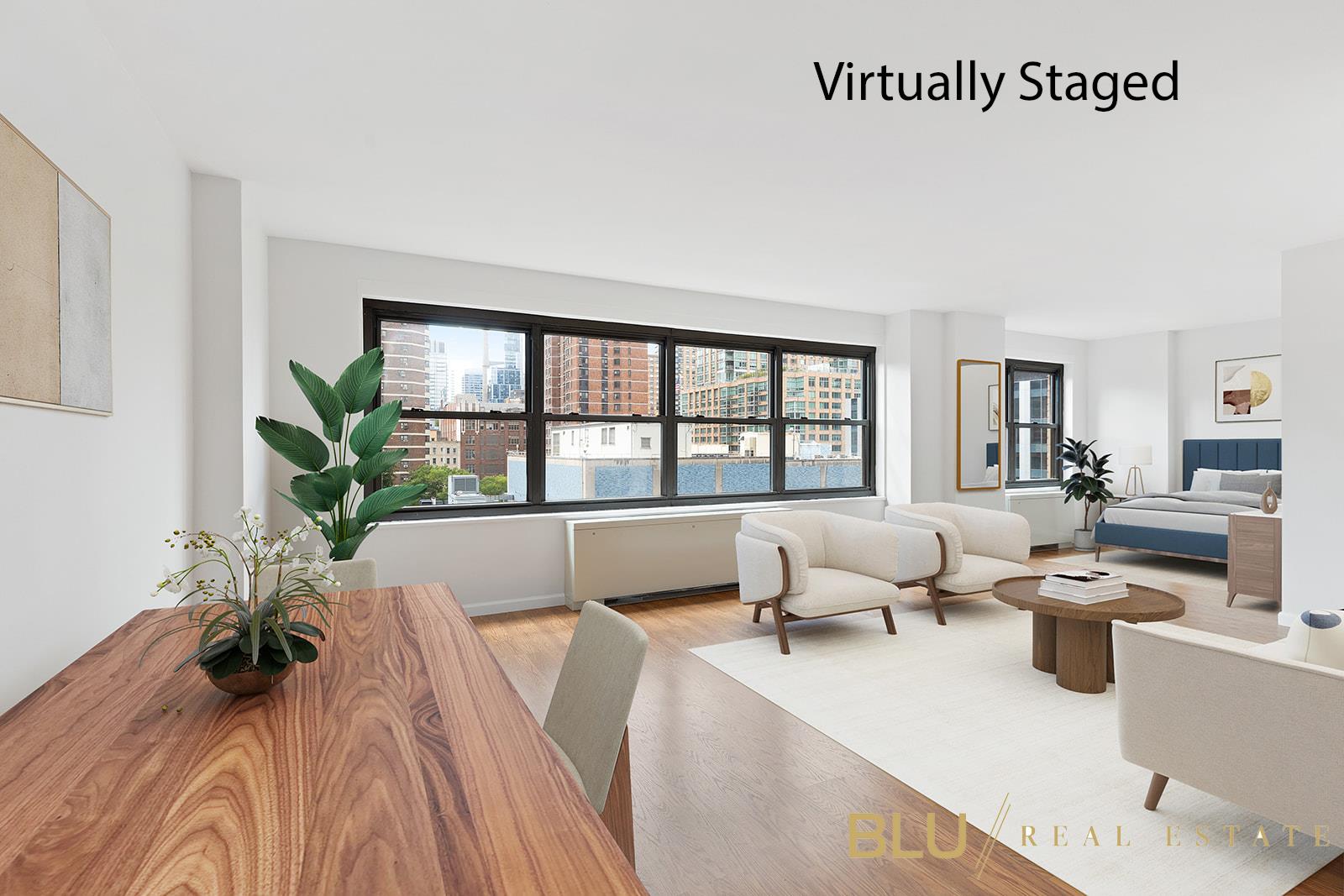The image depicts a well-furnished room with light gray colored walls. On the left wall, there is a framed photograph, mirrored by another framed photograph on the right wall, closer to the bottom left corner. Positioned near the camera is a dark brown wooden table, topped with a small container holding a plant. On the opposite side against the wall, there is a larger plant featuring smooth, teardrop-shaped leaves. The room has hardwood flooring adorned with two chairs that boast large armrests and small legs at the bottom. A round coffee table is placed at the center of a rug, tying the seating area together. On the far side of the room, there is a bed with a blue headboard, flanked by four windows in the middle of the picture, and another window on the right side wall.